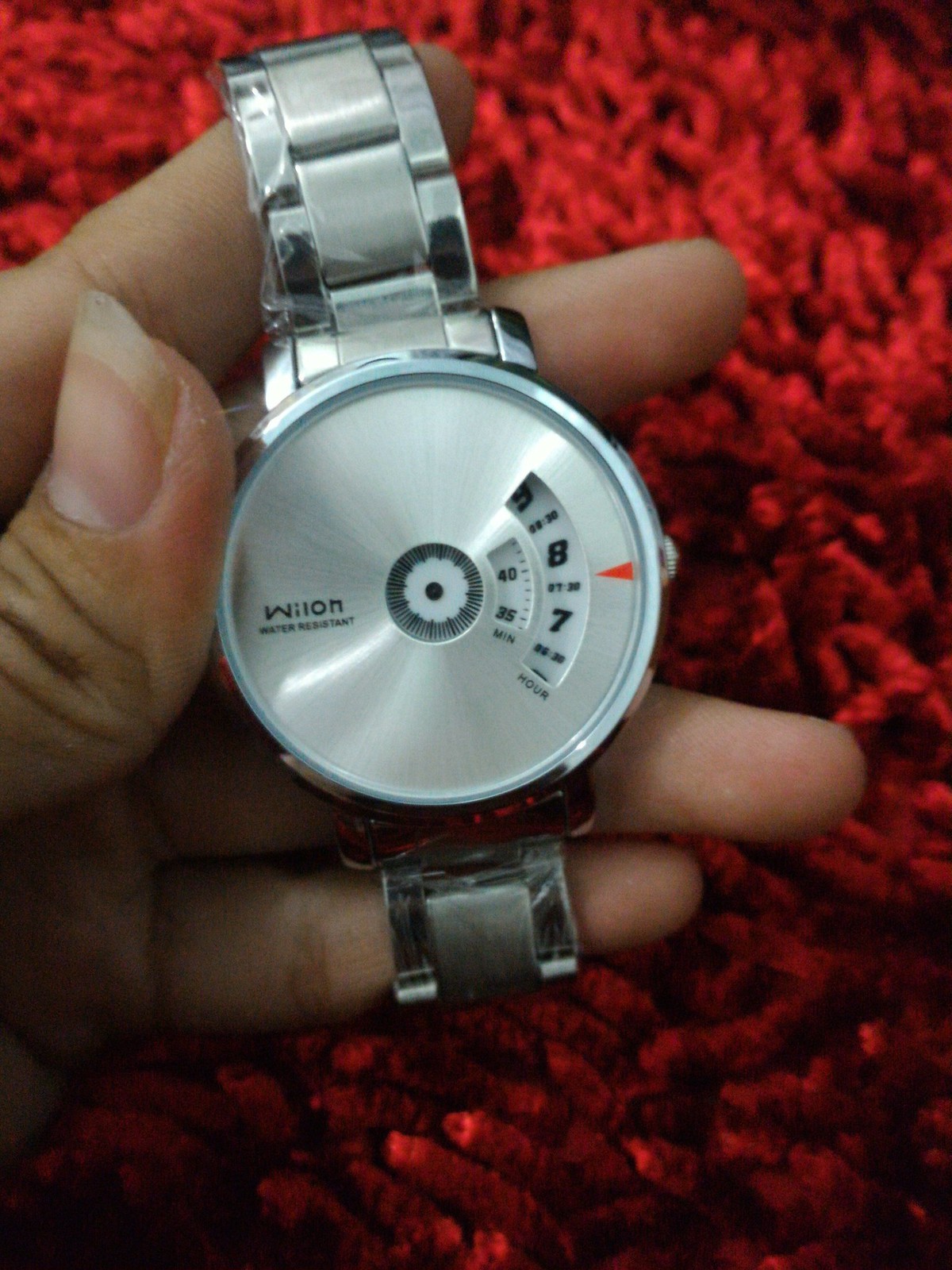In this striking image, a left hand with long fingernails, belonging to a person of fair skin, carefully holds a stylish silver watch. The hand is elegantly poised on a plush, vibrant red carpet that exudes texture and richness. Each of the four fingers is outstretched while the thumb gently curves around the edge of the watch face. The watch itself is a masterpiece; its thick, chain-like strap is made of shiny metal, adding to the overall luxurious look. The watch face features a thin silver rim that slightly protrudes from its surface, which is a polished silver disc. The intricate details include a small golden gear and a white gear on one side, with the brand name "WILON" engraved on the left. On the right side of the watch face are finely-detailed gauges, highlighted by a small red triangle, completing the sophisticated and meticulously-crafted design.